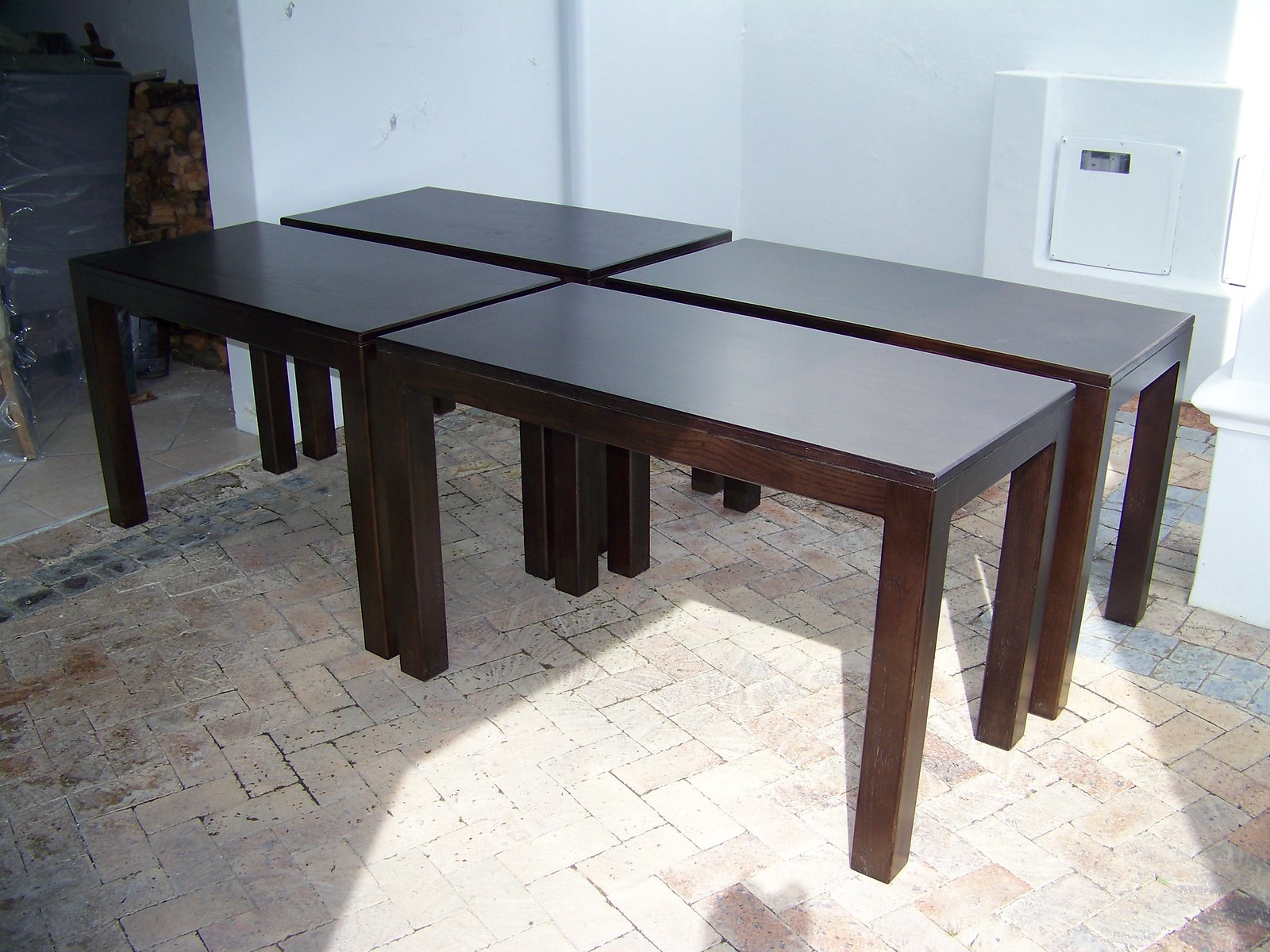This image depicts a room with four rectangular, dark brown wooden tables positioned in the center, pushed together to form a single large table. Each table has four thick, squared legs and a varnished finish. The floor is composed of off-white tiles with a slightly pinkish hue, set in a brick pattern, and shows signs of wear with dark staining in the grout lines. The walls of the room are white, and in the background, there is an open doorway on the left and a small recessed cutout on the right wall that appears to house a fuse box or electrical panel. The image is taken from a side angle, allowing a view of the tops of the tables, which clearly delineates the individual tables by the spaces where they meet, both horizontally and vertically. There is a splodge of sunlight illuminating the lower right corner of the floor.